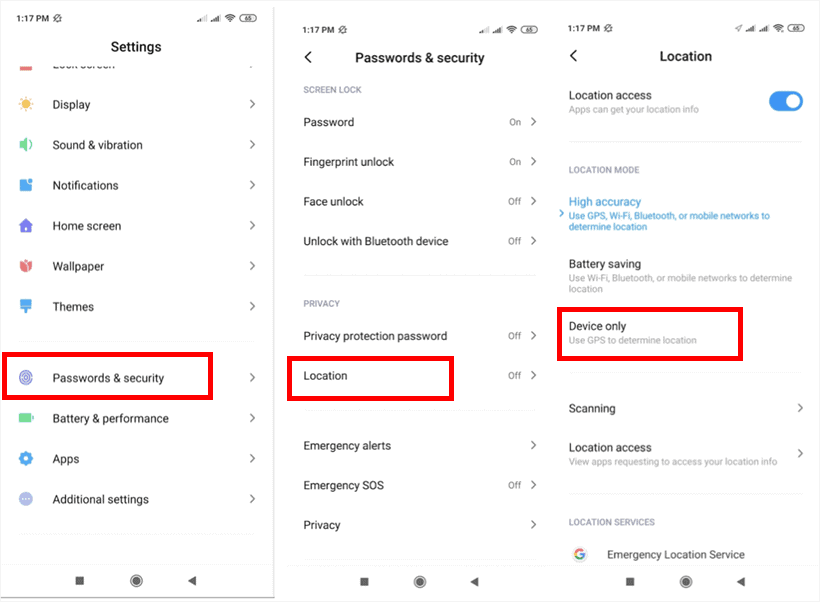This image collage consists of three sequential smartphone screenshots detailing the journey through the device's settings menu, highlighting various security and location settings. 

The **first screenshot** displays the main Settings menu, presenting options such as Display, Sound and Vibration, Notifications, Home Screen, Wallpaper Themes, and Passwords and Security. Notably, "Passwords and Security" is emphasized with a red box, signaling its selection.

The **second screenshot** dives into the "Passwords and Security" settings. Here, we observe that the Screen Lock password is activated, Fingerprint Unlock is on, Face Unlock is turned off, and Bluetooth Unlock is also off. Under the Privacy section, the Privacy Protection Password is disabled, and the Location setting is explicitly marked with a red box despite being turned off, indicating further scrutiny.

Finally, the **third screenshot** focuses on Location settings. Location access is enabled, allowing apps to retrieve location information. The Location Mode options include: 
- **High Accuracy:** Uses GPS, Wi-Fi, Bluetooth, or mobile networks to determine location.
- **Battery Saving:** Utilizes Wi-Fi, Bluetooth, or mobile networks for location data.

The "Device Only" mode, highlighted in a red box, specifies the use of GPS exclusively to determine the device's location, indicating the user's intention to configure location access through this setting.

This series of screenshots documents the user's detailed navigation through their phone’s security and location settings, illustrating their efforts to manage and optimize these features.